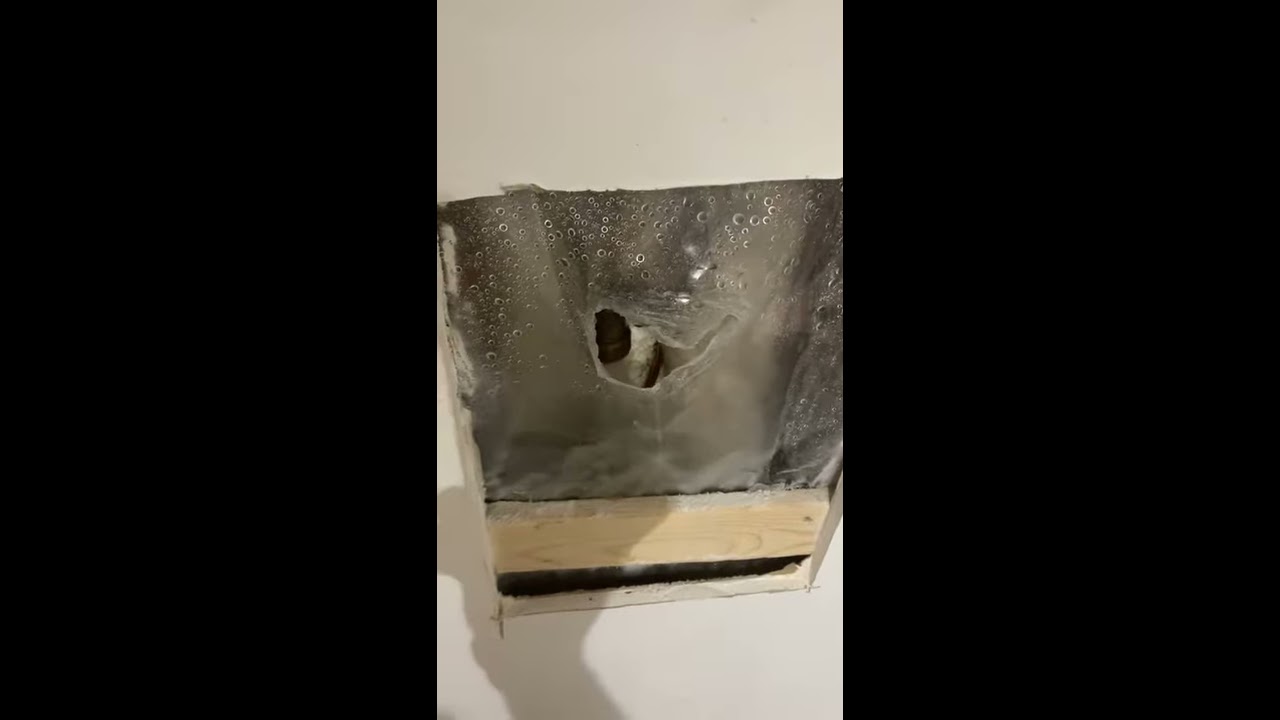In this photograph of an indoor scene, the focal point is a triptych with two wide black panels on the left and right, flanking a central image against an all-white background, including a white wall and floor. The central image prominently features a green canvas knapsack with a triangular hole, positioned within a low crate comprised of a light brown wooden base and two sideboards. The knapsack, which bears white stains and visible water droplets indicating condensation, contains objects that appear to be bottles with black lids and clear liquid. The scene is devoid of text but includes the faint shadow of the photographer, implying an indoor setting. The surrounding elements suggest an amateurish cut in a white drywall, further enhancing the rustic and unfinished aesthetic.